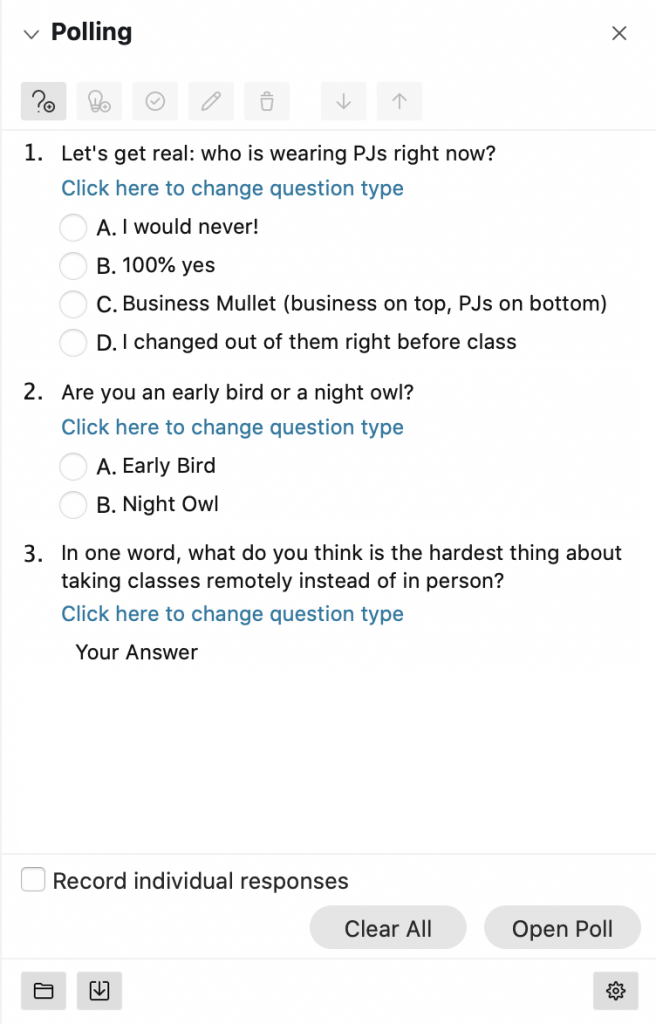Here is a detailed and cleaned-up caption for the image described:

---

This image is a vertical screenshot captured on a mobile device, depicting a poll interface on a white background. A thin vertical gray line runs from the top to the bottom along the left edge, providing a boundary for the poll content. 

In the top section of the screenshot, bold black text in the top left corner reads "Polling," while an "X" icon is visible in the top right corner. Below this header, there are two gray boxes that contain options for editing or deleting the poll, and functionality to scroll through the poll content.

The poll comprises three questions. The first question, listed as "1," asks: "Let's get real, who is wearing PJs right now?" A blue link below the question text says, "Click here to change question type." This question offers four multiple-choice options, each with a radio button:

- A) I would never.
- B) 100% yes.
- C) Business mullet (business on top, PJs on bottom).
- D) I changed out of them right before class.

The second question in the poll is, "Are you an early bird or a night owl?" Again, a blue link stating "Click here to change question type" appears below the question. This question includes two options with radio buttons:

- A) Early bird.
- B) Night owl.

The third and final question prompts the respondent with, "In one word, what do you think is the hardest thing about taking classes remotely instead of in person?" Similar to the previous questions, a blue link below reads, "Click here to change question type." There is a black text input field labeled, "Your answer," where participants can type their response.

At the very bottom of the poll, there is a checkbox beside the text "Record individual responses." Two gray buttons labeled "Clear all" and "Open poll" complete the interface.

---

This caption gives a comprehensive and organized description of the screenshot, detailing the layout and content of the poll.